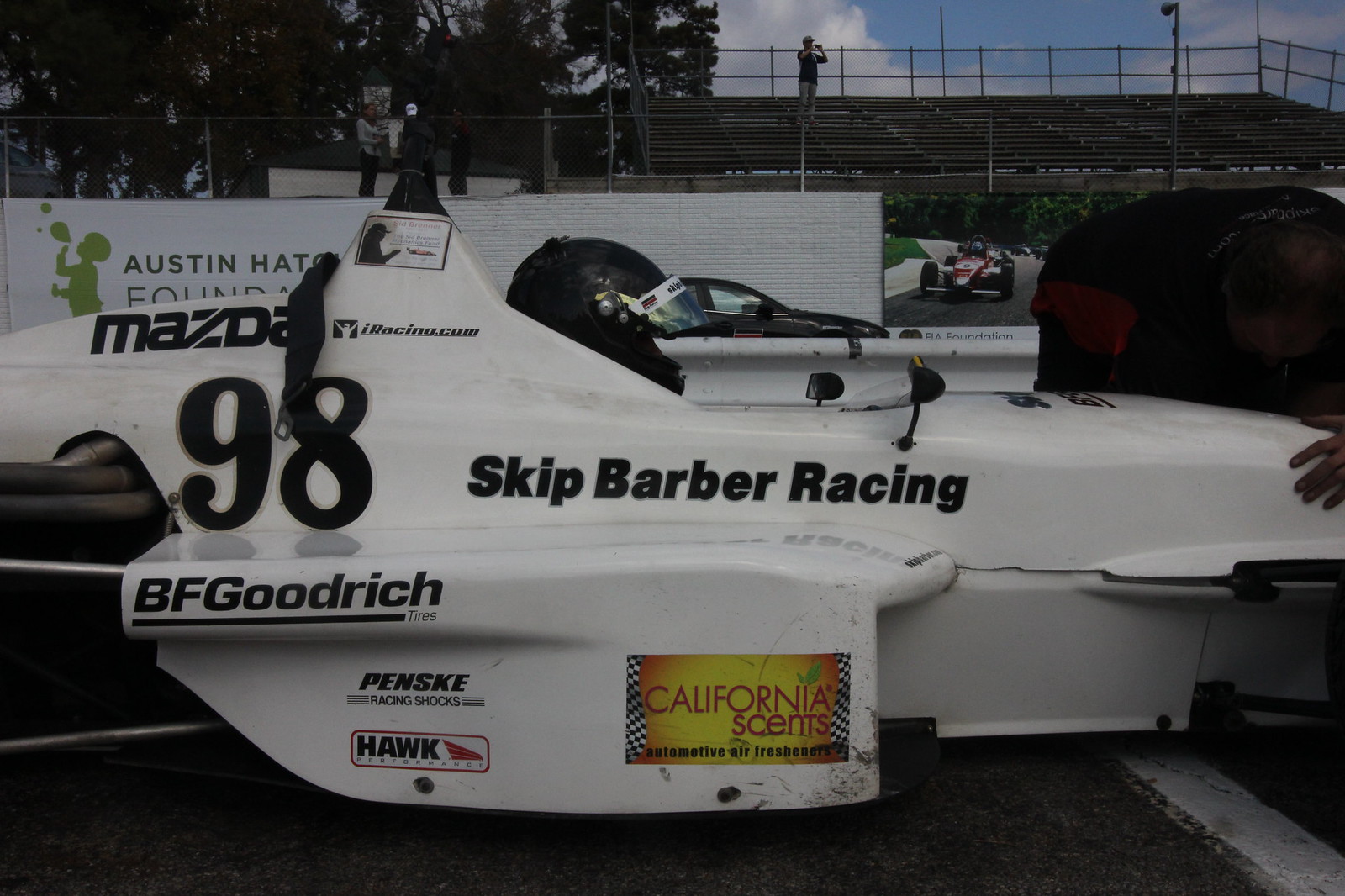The image depicts a close-up side view of a white, unconventionally shaped Formula One race car. The focal point captures the middle of the vehicle, revealing sponsorship logos scattered across its white fiberglass body. Prominently, the back of the car features the black "Mazda" logo and the large number "98." Below the cockpit area, "Skip Barber Racing" is spelled out in black letters, accompanied by additional sponsor logos including BF Goodrich, Penske racing shocks, and California Scents. The cockpit has a driver wearing a black helmet, though their face is partially obscured. A noticeable crack runs through the fiberglass just below the cockpit on the right side of the image. In the background, under a patch of blue sky dotted with clouds, you can see an audience stand with a few people and some trees on the left. On the far side of the car, there is a guardrail with regular cars parked behind it, reinforcing the racing ambiance of the photograph.